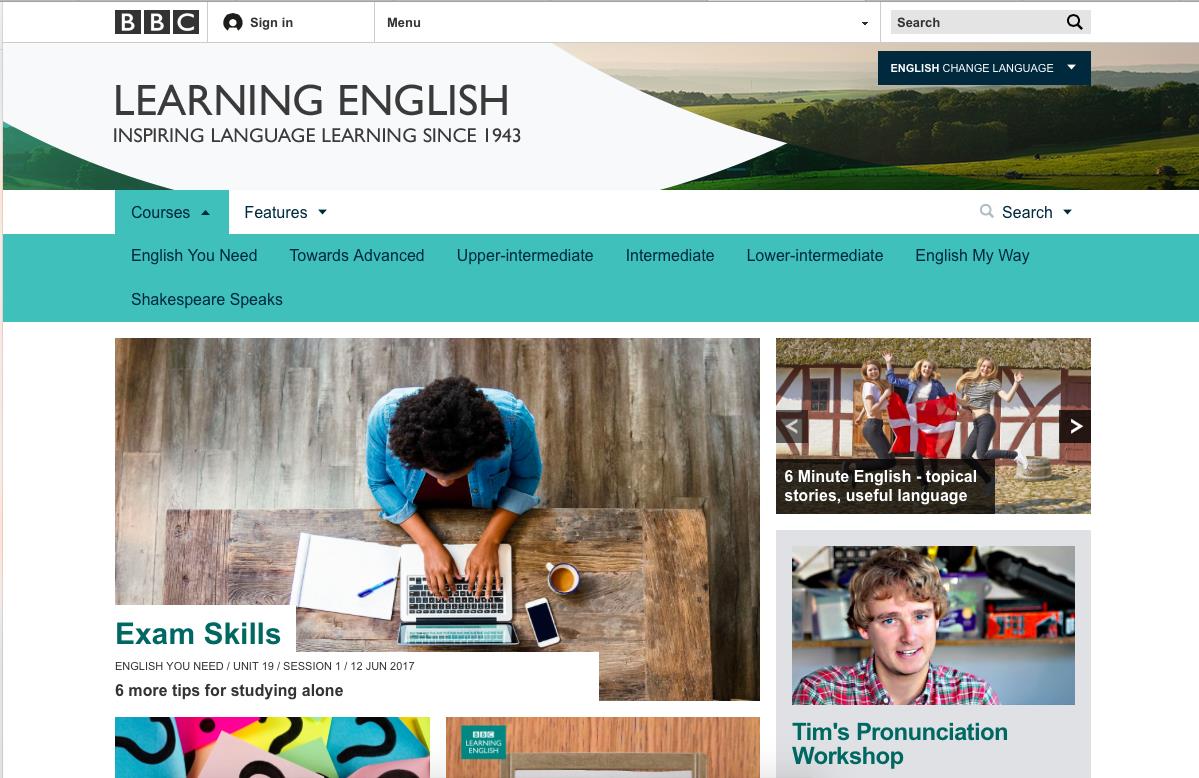This webpage from the BBC is dedicated to language learning. In the upper left corner, there's a "BBC Sign-In" menu, while the upper right corner features a search bar. The main title below these elements, written in all capital letters, reads, "LEARNING ENGLISH. Inspiring language learning since 1943." Directly underneath the title, there's a navigation menu with "Courses" highlighted. Other listed categories include "English You Need," "Towards Advanced," "Upper Intermediate," "Intermediate," "Lower Intermediate," "English My Way," and "Shakespeare Speaks."

The central portion of the page features an overhead photograph depicting a person sitting at a desk, typing on a laptop. On the desk, there is also a cell phone, a cup of coffee, a notepad, and a pen. Underneath this image, the text reads: "Exam Skills. English You Need, Unit 19, Session 1, 12 June 2017. Six More Tips for Studying Alone."

To the right, there's a smaller, outdoor photograph in front of a building, showing three women standing together. One of the women is holding a flag with a red background and a white cross. The caption underneath reads: "Six Minute English. Topical Stories, Useful Language."

Below this, there is a picture of a young man wearing a plaid shirt. The caption under this image simply states: "Tim's Pronunciation Workshop."